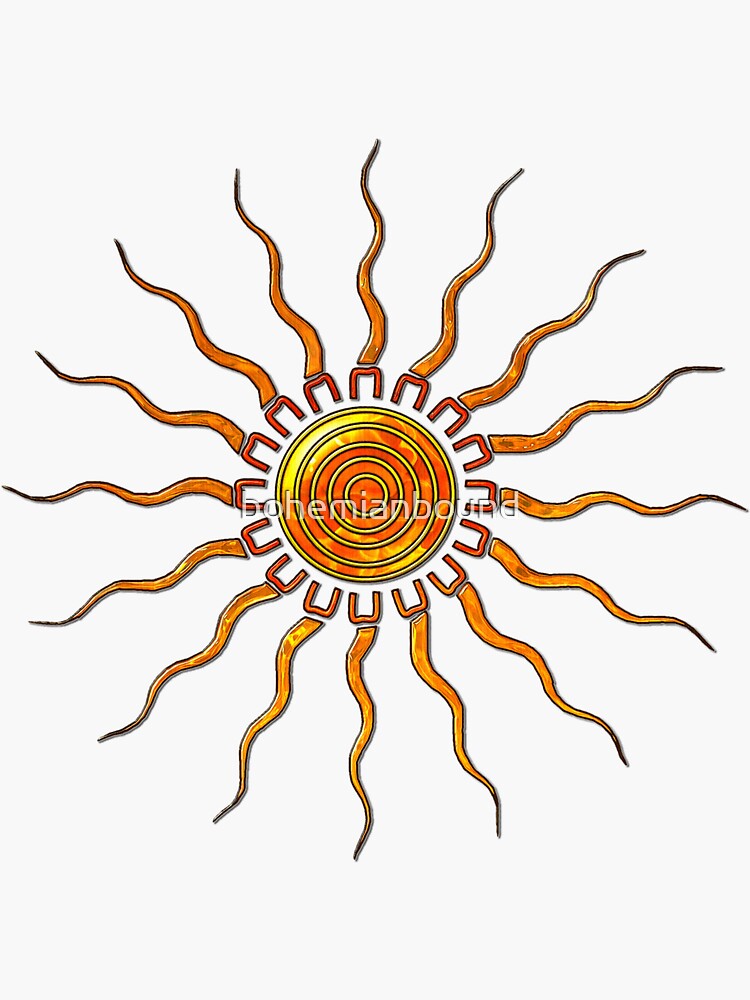The image depicts a stylized sunburst logo, with concentric circles at the center in shades of yellow and orange, resembling swirling smoke. Surrounding these circles are U-shaped, red staple-like patterns radiating outwards, their ends facing inward. From the tops of these shapes extend numerous wavy, squiggly lines in varying shades of orange, representing the rays of the sun. A watermark reading "Bohemian Bound" is subtly imprinted across the very center, in a light, ethereal, and translucent font.